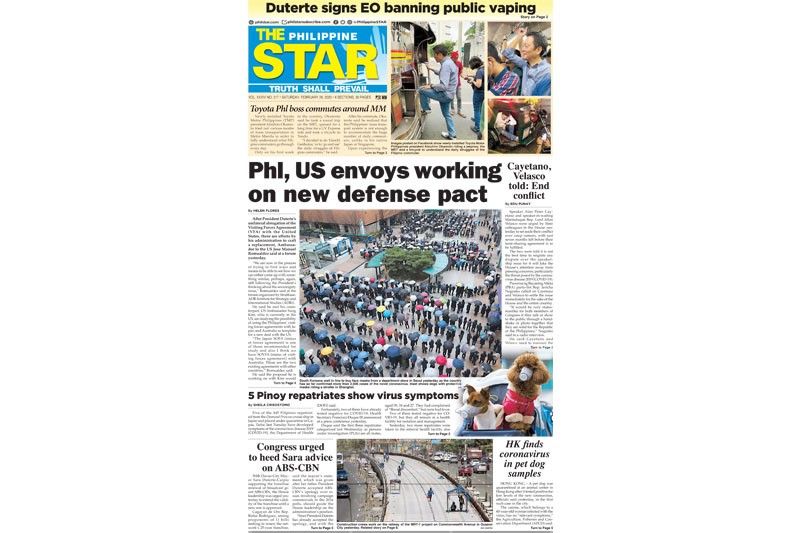In this image, there is a newspaper spread at the top section. The headline features a light brown box with black print that reads "Do you dare to sign EO banning public vaping." To its right, there is a prominent blue box that states "The Philippine Star," with "The Star" in yellow and "Philippines" in white. Below this, a white line proclaims “Truth Shall Prevail” alongside a small sun emblem.

Beneath the headline, there is an article titled, "Toyota Feels the Boss Commutes Around MM." It is set against a light pink background with black text. The article is accompanied by three images: one showing a man in blue boarding a small bus, another of the same man standing in line with his hand raised, and a third showing a man and a boy hugging.

Below these images, another headline says "U.S. on Boys Working on New Defense" and "In Kato the Last Code in Conflict." Dominating the center area, there is a large photo of a crowd of people standing in line. They each have umbrellas and are gathered outside a large building beside a blue-covered area.

Further down, the caption "Bad and Away Repatriate Show Virus Symptoms" can be seen. To the right, there's a notable small image of a baby carriage containing two dogs. The dogs wear masks resembling cups over their noses and are dressed in pink and white outfits, respectively.

Another headline reads "Congress Urged to Heed Sarah’s Advice on ABS-CBN." Adjacent to this, there is a picture of a street with people either walking or running. Lastly, the text "HK Fans Coronavirus and Pet Dog Samples" can be seen.